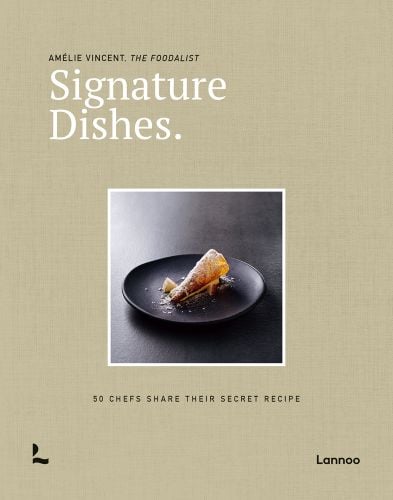This vertical cover image features a minimalist design with a predominantly beige, canvas-like backdrop. At the top, the text reads "Amelie Vincent, The Foodalist" in black font, followed by "Signature Dishes." in larger white font. Centered on the cover is a square photograph with a white border showcasing an artfully presented dish on a black bowl and table, highlighted by angled lighting. The dish appears cylindrical, brown and yellow in color, adorned with white flakes, possibly a dessert. Below the image, in black font, it states, "50 chefs share their secret recipe." In the bottom corners, the publisher's logo and the name "Lannoo" are displayed.